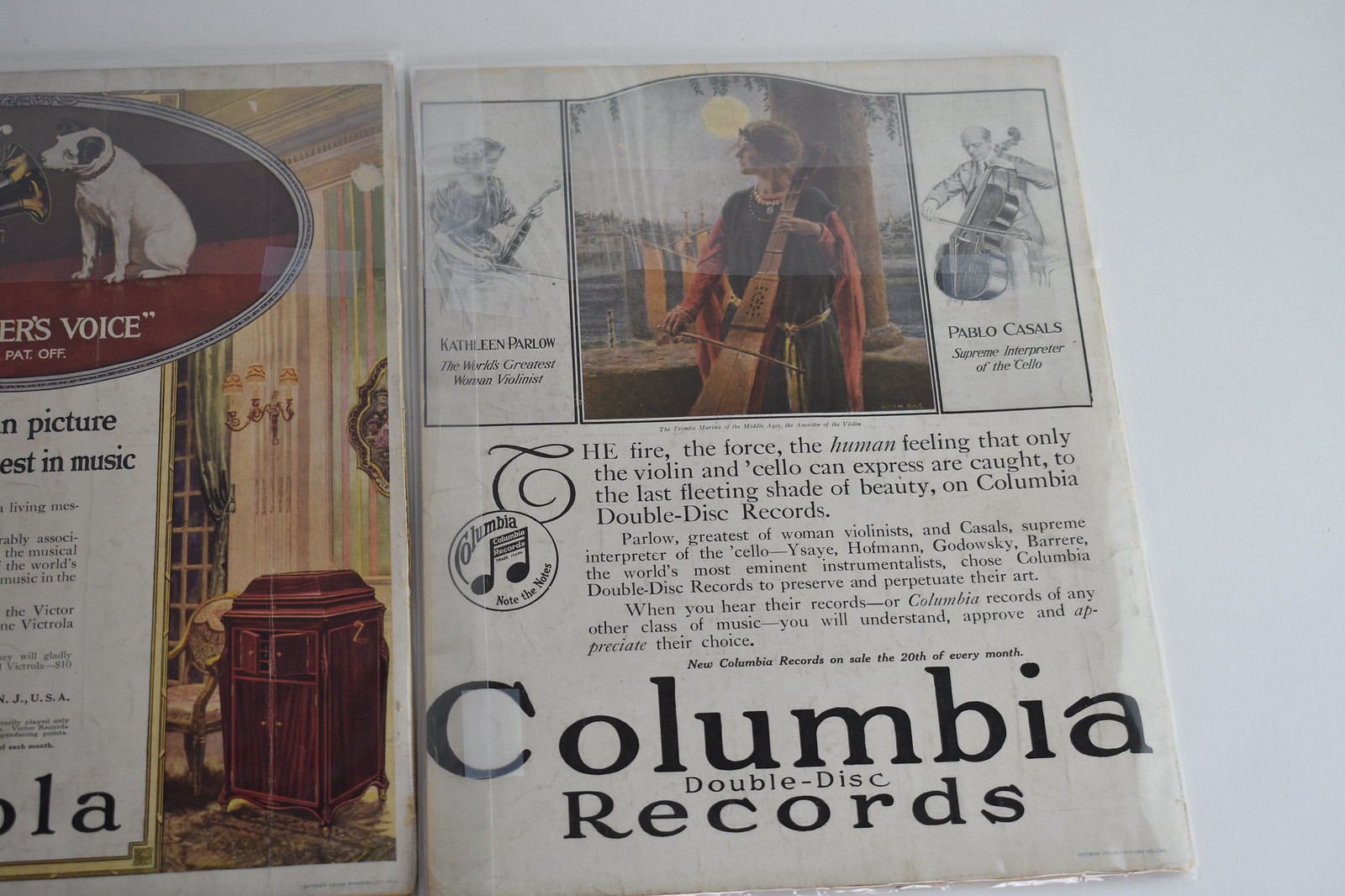This is a horizontal rectangular image resembling a page from a vintage magazine, likely featuring an advertisement. On the right page, there is a picture at the top right corner displaying a woman playing a musical instrument, set against a backdrop of what appears to be a castle-like fortress with a prominent pillar. The image's colors are green and brown, and there is reflected light making it somewhat difficult to see. Adjacent to this image, there is a black and white drawing of a person playing a large bass, identified as Pablo Casals. Another drawing of a woman playing an indiscernible instrument is situated to the left of the main image.

Below this visual array, the text reads: "The fire, the force, the human feeling that only the violin and cello can express. To the last fleeting shade of beauty on Columbia double-disc records." Further down, in large black letters on a white background, it states: "Columbia double-disc records," with "Columbia" appearing in larger font.

On the left page, there is an advertisement featuring the iconic image of a white dog with its face inside a Victrola horn, recognizable as the RCA logo. Below this image, there appears to be an old, large wooden radio set atop a light green rug, placed in a room with brown walls and a big picture window. This page also includes additional text, with visible phrases such as "Picture" and "Music," enhancing the nostalgic ambiance of the scene.